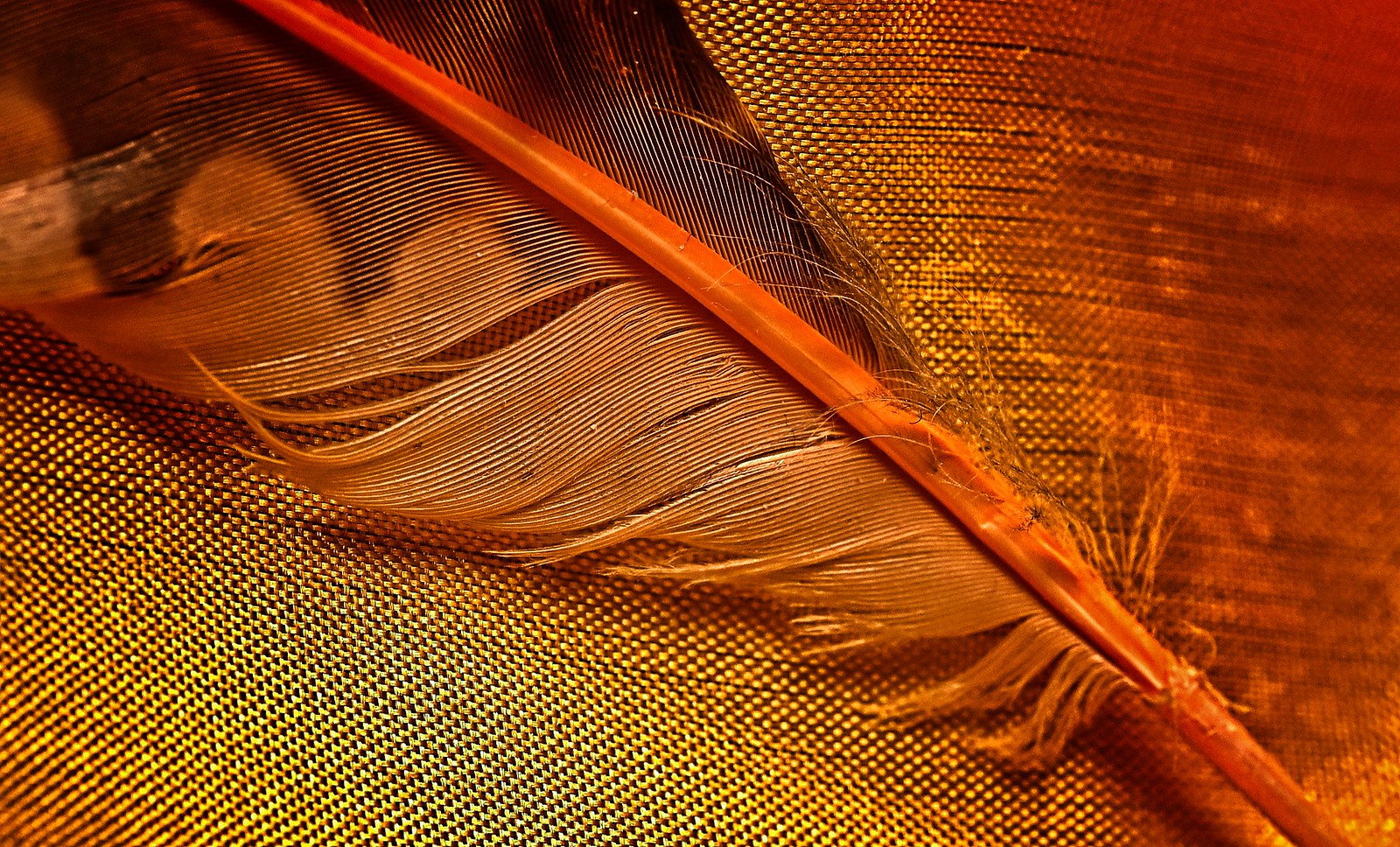This image captures a close-up of a slightly worn and deteriorated feather resting diagonally on a textured piece of cloth with tiny holes. The cloth itself features a gradient of rich colors, predominantly yellows, deep oranges, and dark orangey-reds, with interspersed whites. The background fabric's weave is clearly visible and adds a screen-like quality. The quill of the feather is located in the bottom right corner, extending diagonally to the upper left corner where the feather's larger part goes out of the frame. The feather displays a spectrum of colors including orange, brown, black, and red, with lighter and darker areas interspersed, revealing areas where it is torn or separated. The vein of the feather, prominently colored red, stands out, creating a striking visual against the vivid background. The overall image has an enhanced false color appearance, likely achieved through a gradient color overlay, making the feather and the cloth blend harmoniously in this almost surreal, vibrant orange setting.